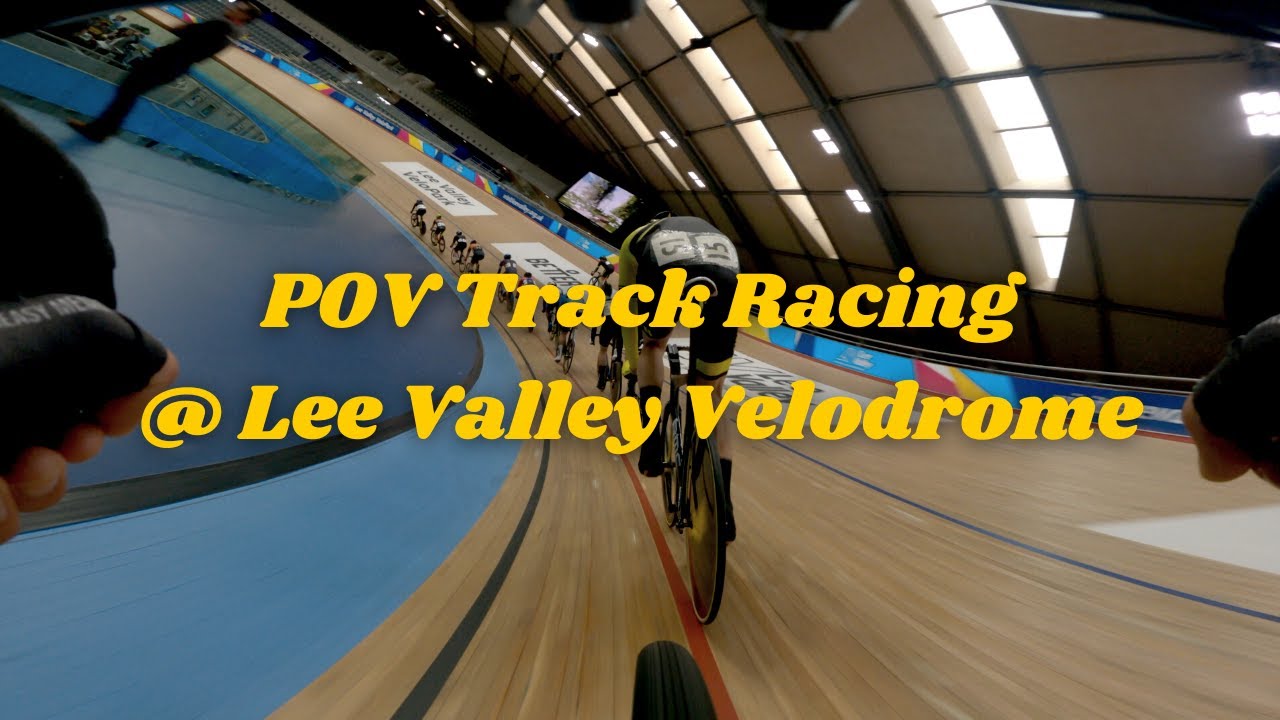This detailed thumbnail captures the exhilarating experience of POV (point of view) track racing at the renowned Lee Valley Velodrome. In this indoor cycling arena, a multitude of cyclists can be seen navigating a circular wooden track under bright ceiling lights. With text written in bright yellow font that reads "POV Track Racing at Lee Valley Velodrome," the image offers a dynamic perspective, as if the viewer is part of the race. The photo is presumably taken from either a video or a GoPro-like device attached to one of the cyclists, providing an immersive feel of the high-speed action. The track is accented with various advertisements, adding to the authenticity of the environment.